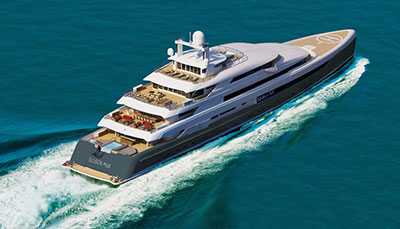This image depicts a sophisticated yacht with three white tiers above its tan main deck, cruising diagonally from the bottom left toward the top right across a calm, blue-green sea. The yacht's design, which could be perceived as potentially CGI or a painting given its video game-like quality, includes a distinct helipad on the extended front deck, outlined by a white circle with a white 'H'. The vessel narrows at the top with a rounded rectangular top compartment featuring six vertically aligned windows and two white orbs supported by a white bar. Foam and turquoise waves generated by the yacht's smooth motion suggest a dynamic, high-speed movement, especially turbulent at the stern. The wraparound railing and multiple decks sport various seating areas, including red chairs, but no passengers are visible.